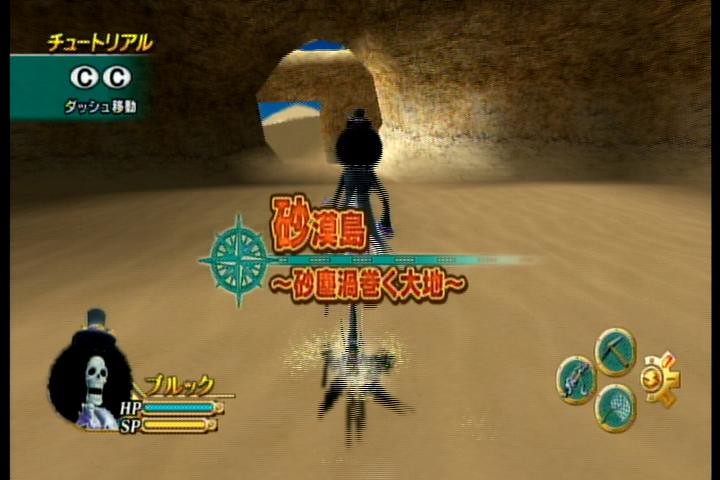In this video game, which appears to be in Chinese, the scene is set in a vast, sandy environment punctuated by two large rock caves. The sky is a clear blue, contrasting with the sandy terrain. In the distance, a hill is visible. A prominent black character with a large round head, long arms, and long legs stands out in the foreground. In the sand, there is also a long, black creature with small legs. At the bottom of the screen, a significant black circle displays a skeletal head icon. There are yellow characters on the screen, along with white text indicating "HP" and "SP."